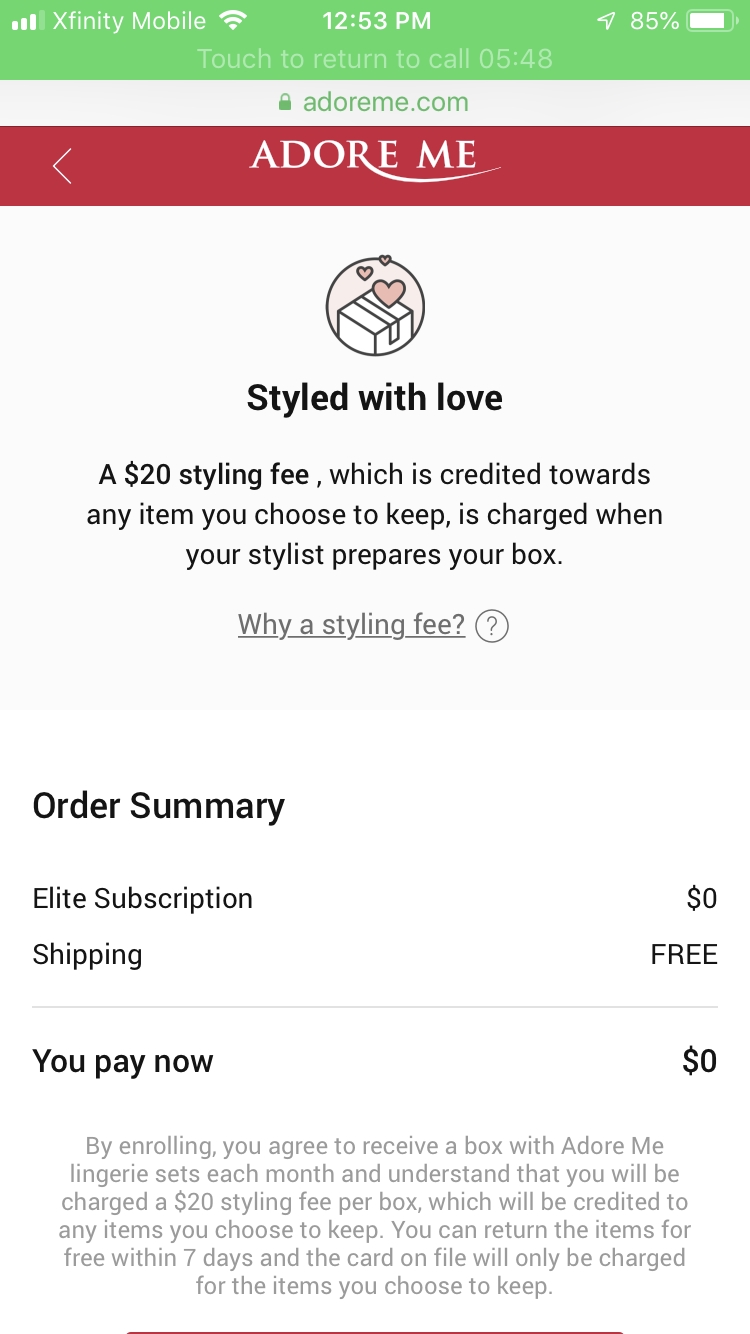This image is a detailed screenshot of the checkout or subscription confirmation page from the Adore Me website, captured at 12:53 p.m., as indicated by the green status bar at the top, which also shows signal strength, Wi-Fi connectivity, and an 85% battery level. The device is connected via Xfinity mobile, with a notification to "touch to return call 548." The URL displayed is AdoreMe.com.

Prominently at the top, a red banner features the Adore Me logo. Directly underneath, a heading titled "Styled With Love" is adorned with icons of a gift box and hearts. The accompanying text explains the $20 styling fee, emphasizing that this fee, credited towards any item kept, is applied when a stylist prepares the box. A hyperlink, "Why a styling fee?", provides additional information.

The image further breaks down the order summary, stating the elite subscription cost is $0, with free shipping. It specifies "You Pay Now" with a total of $0. A disclaimer in smaller text explains that by enrolling, the user agrees to receive a box containing Adore Me lingerie sets each month. It further clarifies that the $20 styling fee per box will be credited towards any kept items, and items can be returned for free within seven days. The card on file will only be charged for items retained by the user.

The layout is designed to inform the user about the styling fee and the cost breakdown before confirming their subscription. Information is clearly conveyed, indicating that while the initial cost is $0, the $20 styling fee (credited towards kept items) will be charged once the stylist prepares the box.